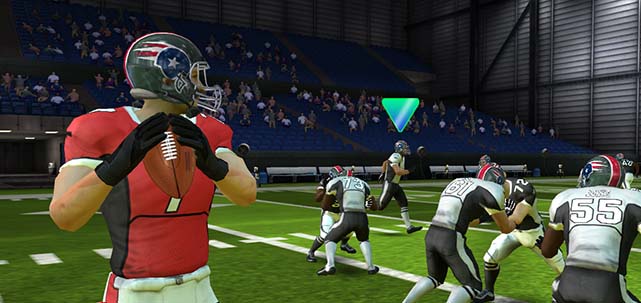This digital color illustration, reminiscent of a modern football video game, is horizontally oriented. It features a football player standing prominently on the left side, wearing a red shirt, black gloves, white pants, and a silver helmet adorned with red, blue, and gray accents. The player is holding a football in front of him. Spread across the middle to the right of the image are several other football players, captured in a dynamic pose as they lean forward and run across the light and dark green field, which is marked with white lines. In the background, there is a stadium filled with blue seats. A steel grid wall encloses the mid and upper portions of the background. An arrow, colored green, white, and blue, is pointing down above one of the players on the field, indicating a specific in-game highlight or focus.